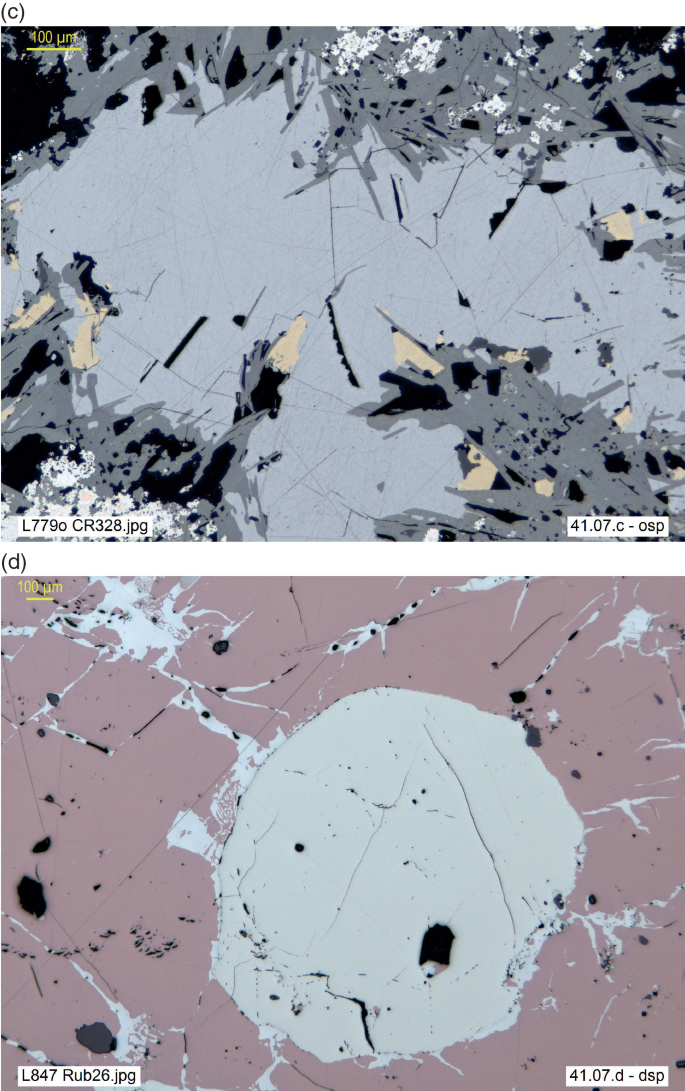The vertical rectangular frame displays two horizontal rectangular images, each occupying the top and bottom halves respectively, resembling maps or aerial shots possibly from a science textbook. The top image, labeled "41.07 C", features a predominantly light gray irregular central area surrounded by darker shades of gray and black with extremely jagged, fractal-like boundaries. The image has accents of tan patches and blue hints, giving it a cracked glass appearance. The bottom image, labeled "41.07 D," showcases a roughly circular light gray area with a violet background, interspersed with gray patterns that resemble rivers or chains of lakes. This image also includes elements described as a pink background and black ink-like blobs, giving it a texture that suggests intergrowths, potentially resembling a skull with a hole in it.